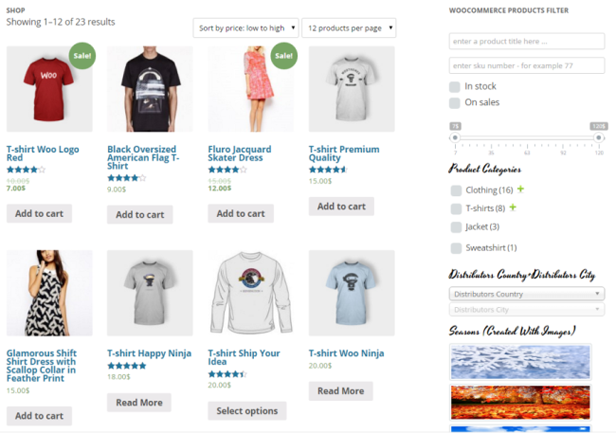Screenshot Description:

The screenshot features an online shop displaying 1 to 12 of 23 results on a white background. The shop utilizes WooCommerce and includes several filtering options. The products are sorted by price, from low to high, with 12 products displayed per page.

1. Red T-Shirt: 
   - Contains a "Woo" logo.
   - Marked with a green circle indicating a sale.

2. Black Oversized American Flag T-Shirt.

3. Floral Jacquard Skater Dress:
   - Marked with a green circle indicating a sale.

4. Premium Quality Glamorous Shift Shirt Dress with a Scallop Collar and Feather Print.

5. Happy Ninja T-Shirt.

6. Ship Your Idea T-Shirt.

7. Woo Ninja T-Shirt.

On the left sidebar, the following categories and filters are visible:
   - "In Stock"
   - "On Sale"
   - "Product Categories"
   - "Clothing" with a subcategory showing 16 items, indicated with a green plus sign.
   - "T-Shirts" with a subcategory showing 8 items, also indicated with a green plus sign.